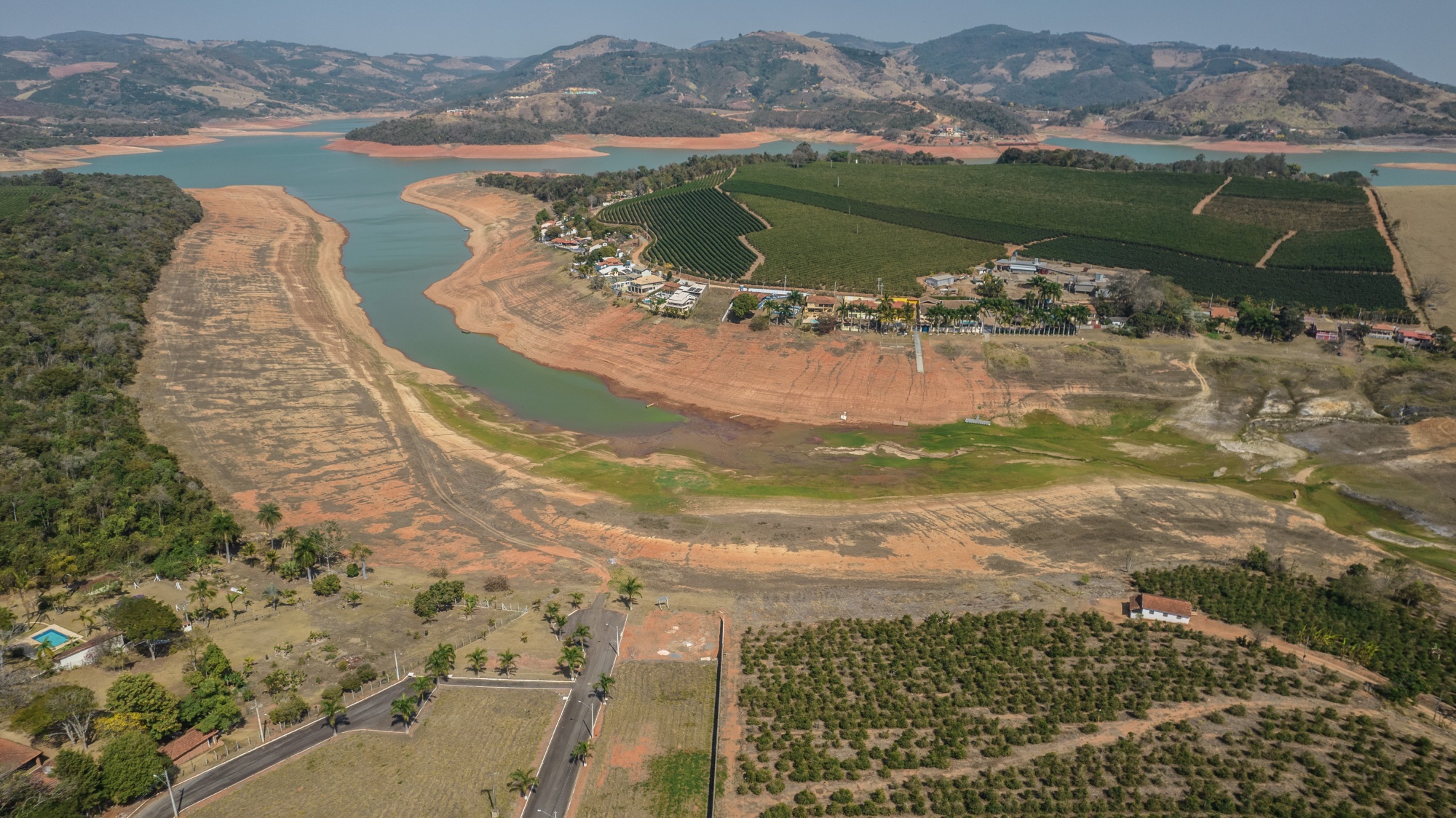This detailed aerial view captures a picturesque lake surrounded by a lush, hilly landscape that transitions from vibrant greenery to rugged, red clay cliffs. The lake's water levels appear low, exposing extensive dirt and banks, which blend into grassy shorelines. The main feature is a small island with minimal housing and buildings, interspersed with cultivated fields and farmlands.

In the foreground, a notable feature is a cultivated area with bushy crops, possibly fruit-bearing, along with a gathering post and pathways. A small house with an adjacent swimming pool is situated nearby. Two meandering gray roadways lead up to the island, enhancing the rural charm of the scene.

The surrounding environment is characterized by green fields, grassy mountains, and a few more isolated houses and restaurants scattered across the landscape. Lampposts dot the roadways, hinting at illumination during nighttime. The sky above is gray and overcast, adding a slightly gloomy ambiance to this serene natural setting.